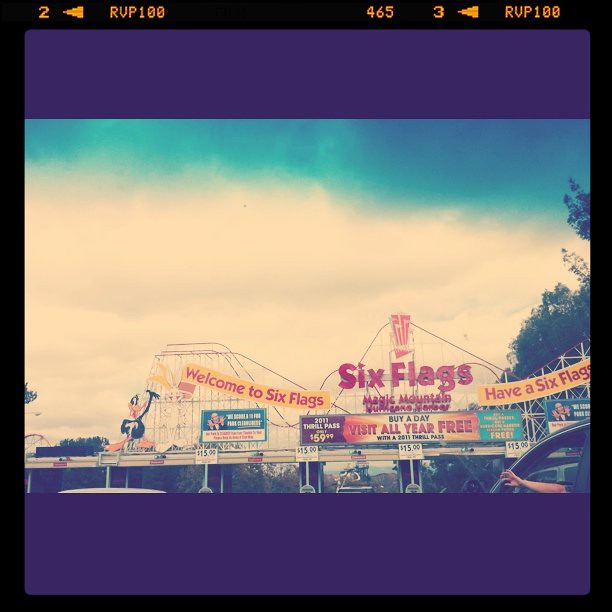This image depicts the front entrance of Six Flags Magic Mountain, with visual elements suggesting it's an older photograph. Dominating the top of the image is a black-bordered banner featuring orange text: on the left, the number 2 followed by a left-pointing arrow and "RVP 100," and on the right, the number 465 followed by a space, then a 3, a left-pointing arrow, and "RVP 100" again. The image features a purple border at the top and bottom, a blue but cloudy sky, and various signs with pricing information. One sign promotes a "2011 Thrill Pass" for $59.99, which offers all-year access for the price of a single day's visit. Another sign displays the price "$15.00."

In the foreground, partially cut off, text reads "Welcome to Six Flags, have a Six Flags," with "Magic Mountain" also visible. To the far left, Daffy Duck is present, characterized by his black body and bill. Additionally, the iconic Old Man from Six Flags seems to be here, although this caption might be a bit unclear. A large roller coaster stretches across the background, reinforcing the theme park setting, with a bit more visible on the left. At the bottom right, a hand extends from a car, signaling for the car behind to wait.